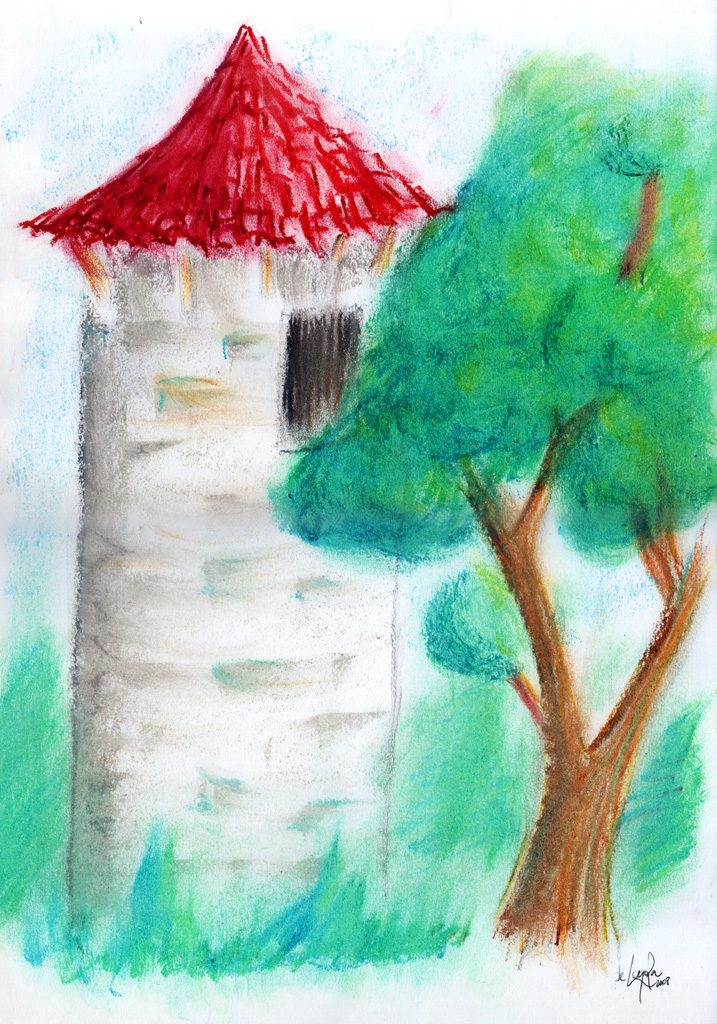The image depicts a detailed sketch of an imposing, castle-like house characterized by its tall and slender white facade, almost resembling an elongated oval or rectangular shape. The structure is capped with a vibrant red roof, lending a dash of color contrast. A single, dark window punctuates the otherwise smooth outer wall, with ominous black bars adding an element of intrigue or security.

In the foreground, there's a carefully sketched tree, which stands in stark contrast to the house. Its trunk and branches are rendered in shades of brown and orange, while the foliage is lush green. At the base of this scene, tufts of green grass appear to encroach upon the house, adding a touch of nature reclaiming space. The whole composition is a harmonious blend of architectural and natural elements, brought to life through intricate sketchwork.